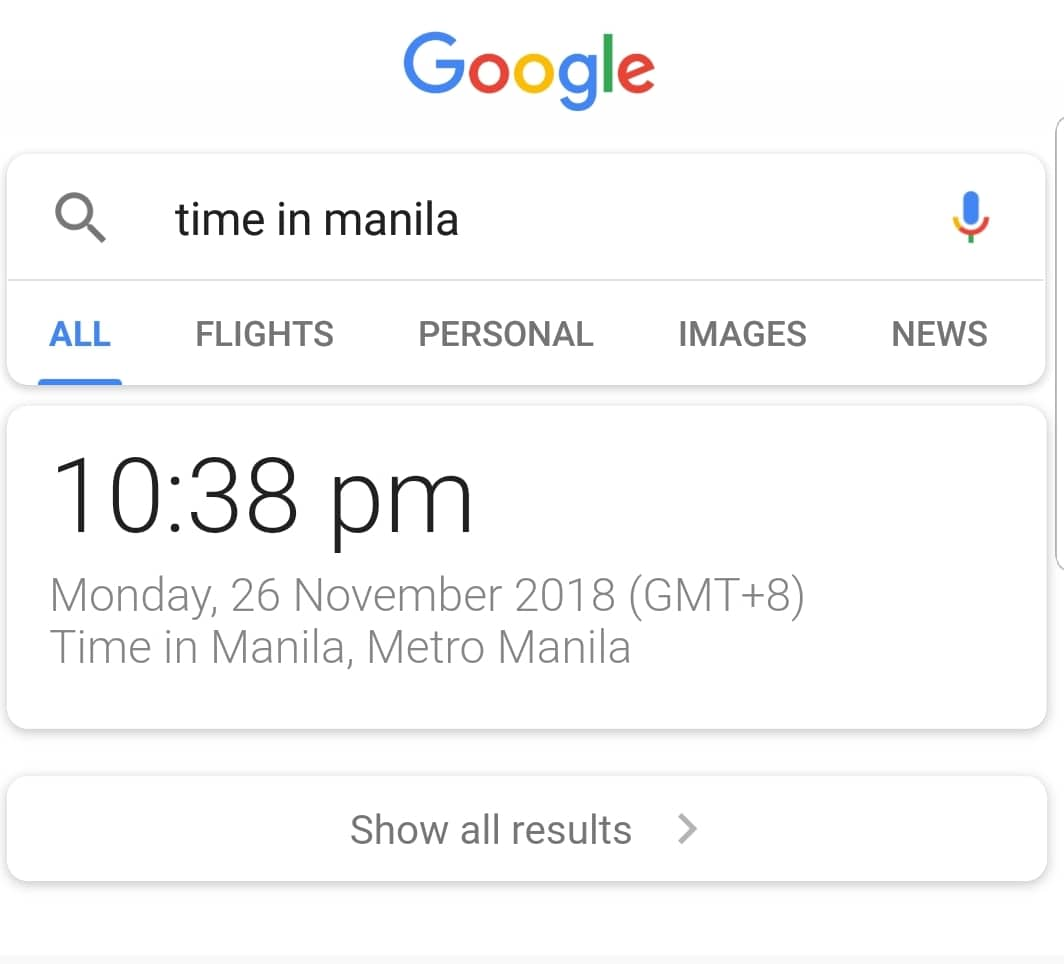In the top center of the image is the iconic Google logo, featuring a capitalized blue 'G', followed by 'o' in red, 'o' in yellow, 'g' in blue, 'l' in green, and 'e' in red. Below the logo, a search bar filled with the query "Time in Manila" is prominently displayed. To the left of the search bar, there is a magnifying glass icon symbolizing the search function, while to the right, a colorful microphone icon in blue, red, yellow, and green indicates voice search capability. 

A dividing line separates the search bar from the five navigation links underneath: 'All', 'Flights', 'Personal', 'Images', and 'News'. The 'All' link is highlighted in blue, signifying it's the current selection, while the other links are styled in red. 

Beneath these links, in a separate white box, the current time in Manila is displayed as "10:38 PM" in gray text. Below the time, the date "Monday, 26 November 2018" is subtly noted, providing clear and precise information about the local time and date.